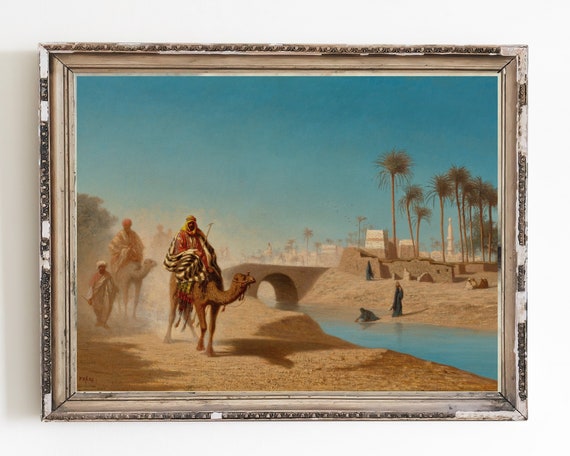The square image depicts a framed piece of art mounted or leaning against a light gray or white wall. The frame itself is made of distressed wood with a light brown and silver finish, and has decorated raised edges, giving it an antique appearance. The artwork within the frame portrays a vivid desert scene. The background features a clear blue sky at the top, complementing a narrow, blue river or stream that runs diagonally from the lower right corner towards the left side. A light-colored bridge spans the river, linking the left and right sections of the scene.

On the right side of the image, there's a cluster of tall palm trees and two people near the river's edge—one leaning over the water and another standing behind them, both appearing as black outlines. On the left side, two men wearing robes and head coverings ride camels, facing towards the viewer. Alongside them, another man walks on the sandy ground. The sandy foreground extends throughout the scene, and in the distant background, more palm trees and buildings are visible, adding to the depth and richness of the desert setting. The overall image is bright and clear, signifying a well-lit environment.